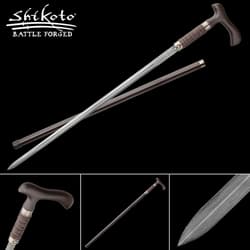The image features an advertisement for Shikoto Battle Forged, displayed prominently in white lettering at the upper left corner. Set against a black and gray background, the focal point is a weapon that appears to be a disguised sword, resembling a walking cane. The cane handle, made of dark-colored wood with a T-shaped design, is positioned in the bottom right corner of the image. The cane itself is diagonally arranged from the bottom left to the upper right, showing the top part removed to reveal a thin, silver, sword-like blade. The sheath, or bottom part of the cane, is metal and pointed at the end, indicating its dual purpose. The casing features a blend of brown and gold hues, further enhancing its intricate design.